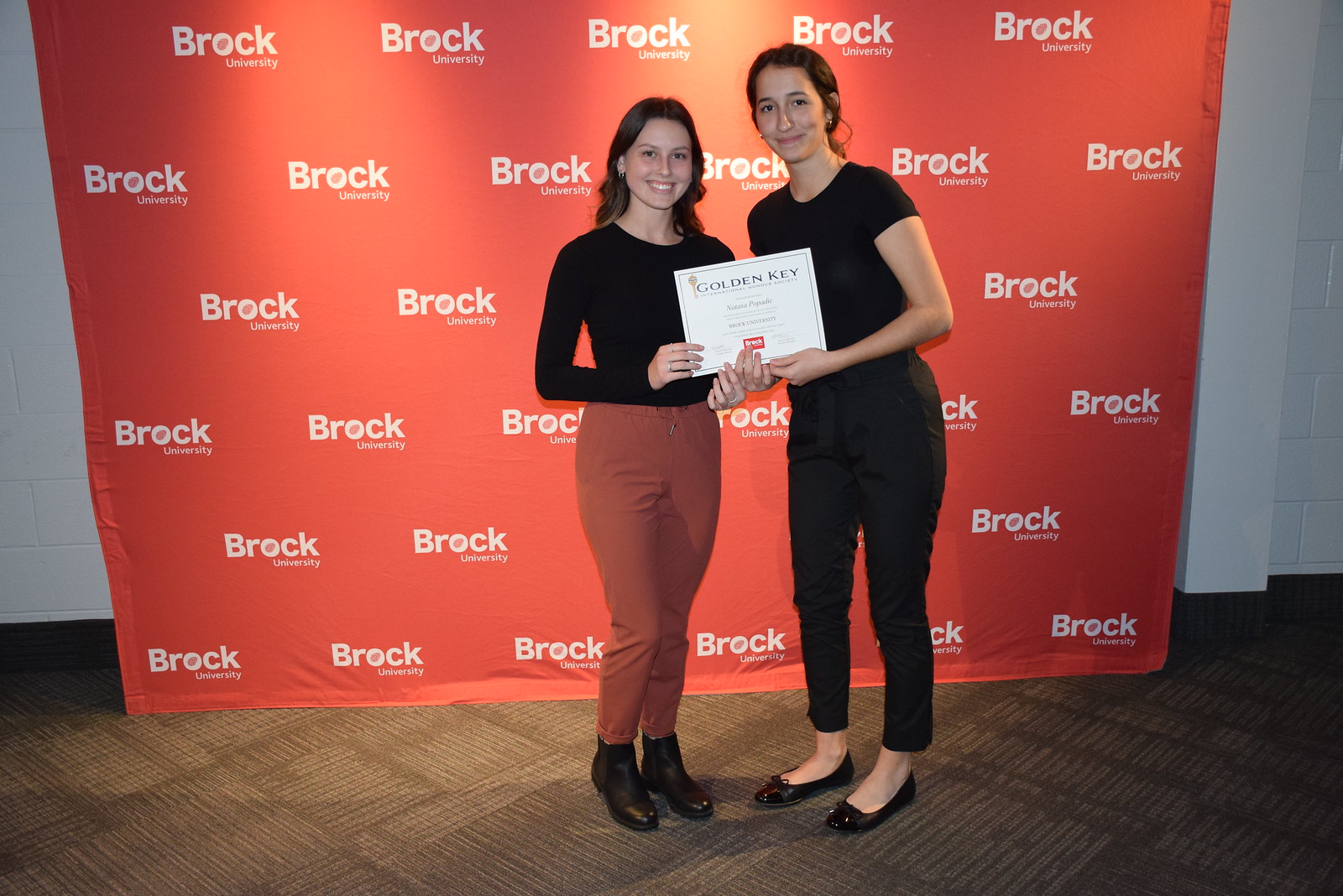In this photograph, two smiling women stand on brown and beige carpet against a vibrant orange-red backdrop adorned with the white text "Brock University," repeated in a tile-like pattern. The woman on the left has long brunette hair and wears a dark long-sleeve blouse paired with pinkish-maroon dress pants and black boots. She holds a certificate jointly with the woman on her right, who has brown hair styled in a ponytail, and is dressed in a black short-sleeve top, black dress pants, and black flats. The certificate they hold prominently features the words "Golden Key." The taller woman slightly bends down while they both face the camera, creating a warm and celebratory moment captured in the photograph.